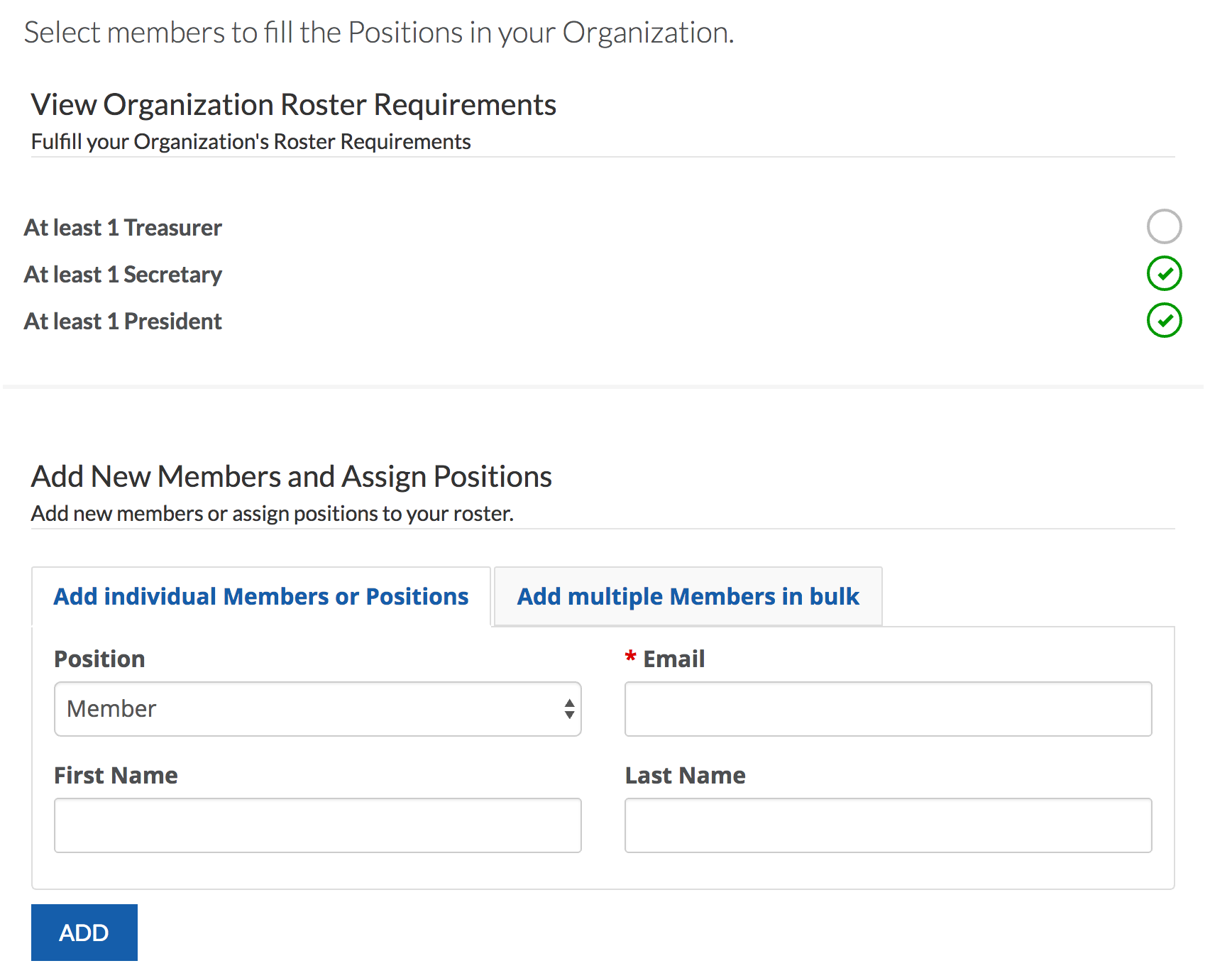The image's background is predominantly white, with significant details highlighted in black text. On the left-hand side, there's a directive that reads: "Select Members to Fill the Position in Your Organization." Further down, the text lists options: "View Organization Roster Requirements," and "Fill Your Organization's Roster Requirements." Specific role requirements are outlined as needing at least one treasurer, one secretary, and one president. 

Adjacent to this, on the right-hand side, are three circles numbered 4, 3. The first circle appears empty, while the last two circles contain green checkmarks, indicating that the positions of secretary and president are filled.

Below this section, instructions in black text state, "Add New Members and Assign Positions." There are two tabs; the white tab on the left is labeled "Add New Members or Positions," and the gray tab on the right says "Add Multiple Members in Bulk." 

Further instruction boxes prompt: "Position," with a dropdown menu to select a member, followed by "First Name," with a text box filled in. An email section is marked by a red asterisk indicating a required field, but the accompanying text box is empty. Similarly, a "Last Name" field is present with an empty text box below the email field.

On the left side of this layout, there is a prominent blue rectangle button with the word "Add" written in white text.

This detailed image guides users on how to manage and fill required organizational roles by adding new members and assigning them to designated positions.